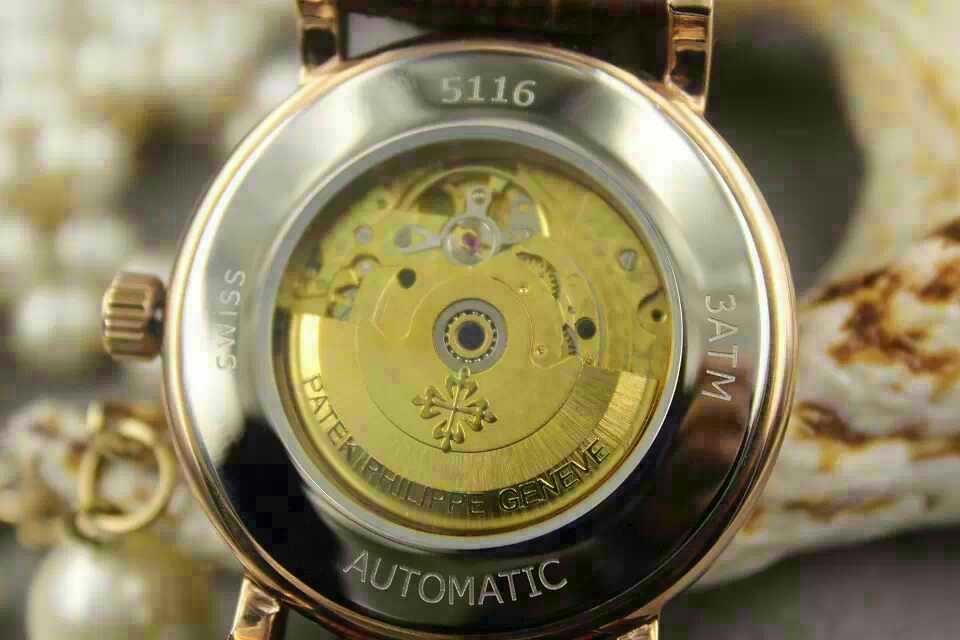This image showcases the intricate back view of a Swiss-made automatic watch. The timepiece displays exquisite craftsmanship through its exposed mechanism, revealing gold-toned gears and dials that interlock seamlessly to measure time. The silver backplate of the watch is elegantly engraved with notable inscriptions, including "Swiss Made" and "Automatic," as well as a partially visible patent reference, hinting at its precision engineering. The watch's winding spindle, used to set the time, is prominently visible. The overall setting presents the watch against a background that appears to be a pearl necklace with hints of brown, adding a touch of sophistication to the scene.